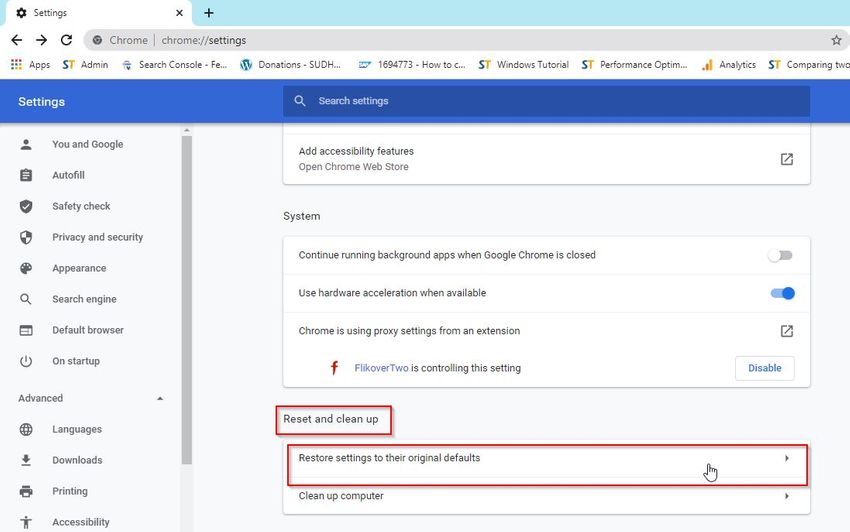The image displays a section of Google Chrome's settings interface. At the top is the address bar showing the URL: "chrome://settings." Below the URL, the settings options are listed in a column, each written in black. The categories include "You and Google," "Autofill," "Safety Check," "Privacy and Security," "Appearance," "Search Engine," "Default Browser," and "On Startup." Further down, under an expandable section titled "Advanced," the options include "Languages," "Downloads," "Printing," and "Accessibility." Above these options, a blue bar extends horizontally across the screen. On the left end of the bar, the word "Settings" is displayed, while toward the center it says "Search Settings." Additionally, a segment above the options displays entries such as "Apps," "Admin," "Search Console," "F.E. Donations," "SUDH," "1694773-howto," "Windows Tutorial," "Performance Option," "Analytics," and "Comparing To."